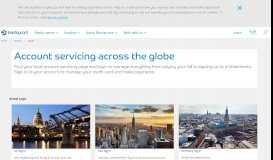The image features a compact screen with tiny, barely legible text. Central to the screen is a blue text that reads "Account Servicing Across the Globe." The top of the image contains a brief text segment on a light gray background spanning the width of the image. Below this is a white section divided into four categories, followed by another light gray strip. Surrounding the central "Account Servicing Across the Globe" text is a white background with an additional sentence beneath it. 

At the bottom of the image, there are three photos. The left photo showcases a cityscape with water in the foreground and a clear blue sky. The middle photo provides an aerial view of a city with skyscrapers. The right photo is another view of a city with tall buildings. On the far right side of the image is a narrow black bar running from top to bottom, serving as a divider.